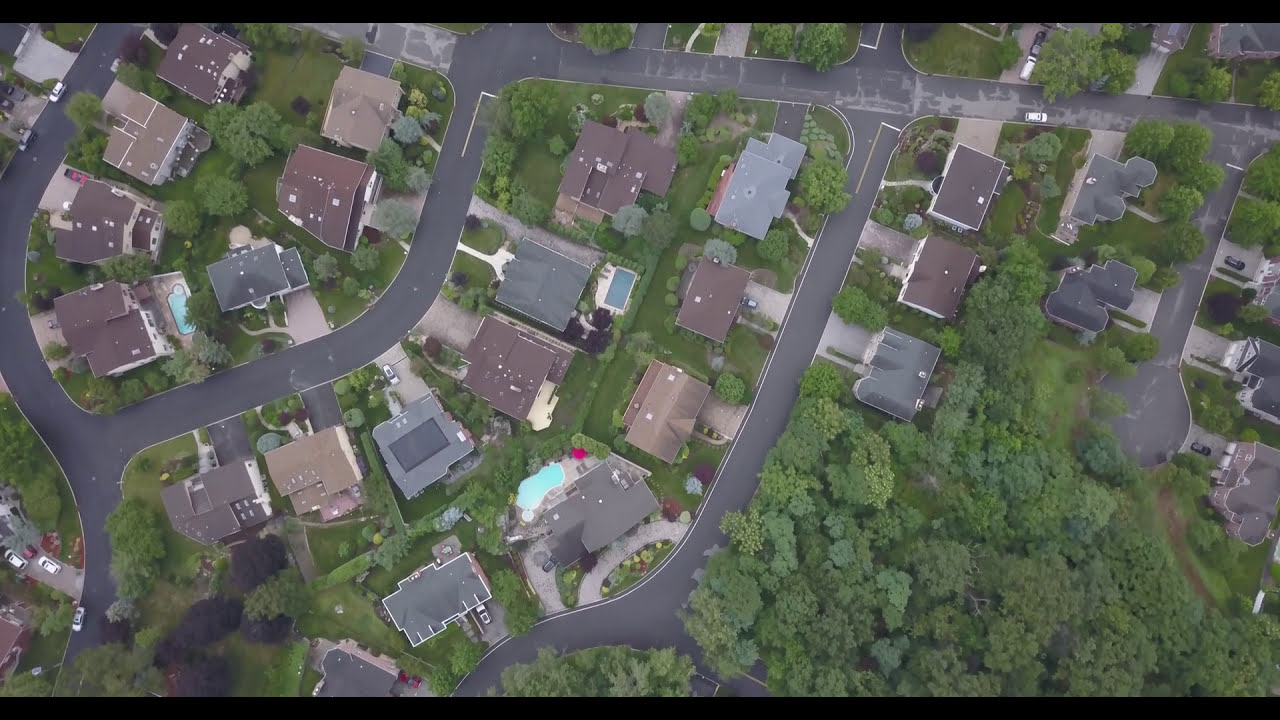This top-down aerial photograph captures a detailed view of a planned residential neighborhood. At the top of the image, a wide black paved road forms the main artery, extending downward with three substantial streets branching off. The street on the right terminates in a cul-de-sac, while the center street continues all the way down to a circular road at the bottom. To the left, a street branches downward before looping back up in a Y-shape. Additionally, there's another road at the bottom of the image. The area is densely populated with large residential houses, predominantly featuring brown and some gray rooftops. Notably, at least one house is equipped with solar panels and two homes have swimming pools in their backyards. The development is lush with green trees scattered throughout, enhancing the suburban aesthetic. The layout resembles a life-sized version of a children's play mat, where roads wind and curve around seamlessly.